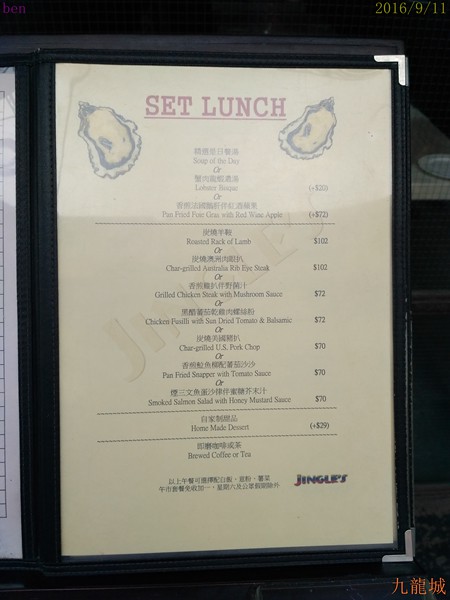The image depicts a menu that is dated September 11, 2016. The menu appears to be behind a glass pane, suggested by the presence of some striping that looks like reflections on glass. Additionally, the composition might include the partial view of a seat or someone holding the menu, though these elements are not clearly discernible.

The menu itself is bi-fold, resembling an open book, and is encased in black with a protective plastic cover. Unfortunately, the left side of the menu is almost entirely cropped out, offering only a sliver of visibility. The right page of the menu is more legible and features various details.

At the bottom right corner of this page, the word "Jingles" is prominently displayed, likely indicating the name of the establishment. The menu's background is off-white, accentuated by large red letters at the top that read "Set Lunch." The upper section of the page includes two hand-drawn illustrations of food items, whose specific details are indeterminate.

The menu features text in both an unspecified Asian language and English. The English section lists various dishes and beverages, including chargrilled U.S. pork chop, roasted rack of lamb, ribeye steak, grilled chicken steak with mushroom sauce, homemade dessert, brewed coffee, and tea. Prices for these items are noted on the right side of the page.